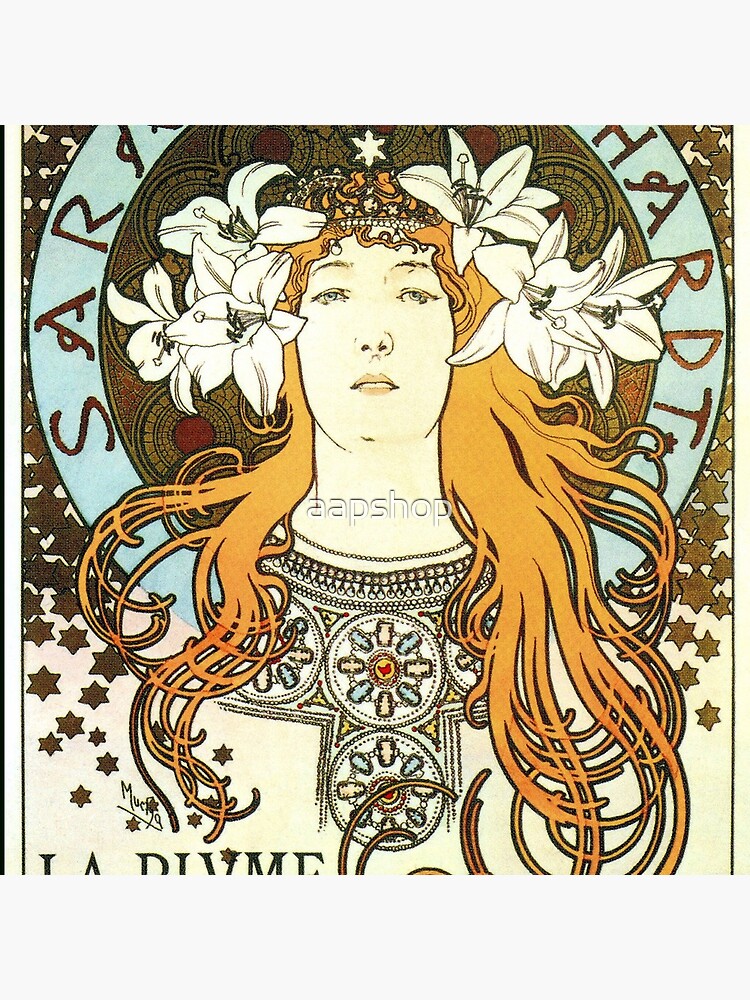The image is a highly detailed poster illustration featuring a white woman with long, flowing gold hair. She is adorned with a crown and white flowers, likely orchids or irises, on each side of her head. The centerpiece of her forehead displays a star, with additional stars surrounding her head. The woman's attire is intricately decorated with various multi-colored necklaces and rounded emblems on her dress, which include white, yellow, and other hues. Among these emblems, there is a small red object that could be a heart or a stylized piece of jewelry. Surrounding her is a design comprising blue, gold, and red ornaments, and the entire image is framed by a decorative blue emblem marked by brown stars at the outer edges. The text on the poster includes a barely discernible name, possibly "Sarah Hart," and the words "AAP Shop." The overall aesthetic of the poster hints at a 'flower woman' or 'hippie' theme, enhanced by the floral arrangements and symbolic elements in her attire.